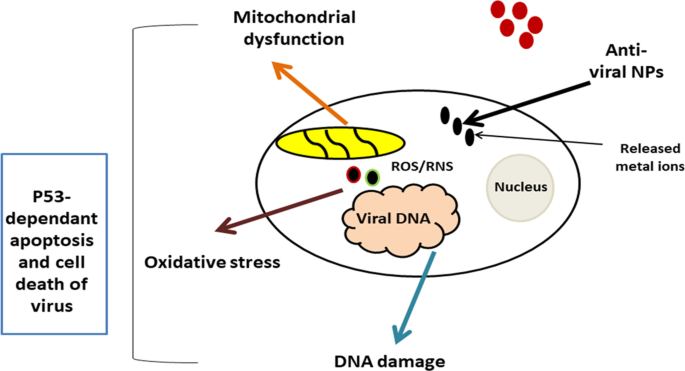This detailed chart is labeled "P53-dependent apoptosis and cell death of virus" and illustrates various biological processes. The central feature of the illustration is a large, sideways oval resembling an egg. Inside this main oval, multiple labeled components are interconnected with arrows. At the top, three black dots marked "antiviral NPs" are connected by an arrow reading "released metal ions." Within the oval, a gray circle labeled "nucleus" is adjacent to a peach-colored, cloud-like structure labeled "viral DNA," from which a blue arrow indicating "DNA damage" extends outward.

Nearby, two small circles—one red with a black center and one green with a black center—are marked with an arrow labeled "oxidative stress." Also inside the oval is a yellow oval with three squiggly lines, marked "mitochondrial dysfunction." In the center of the main oval are the letters "ROS/RNS." Surrounding the main oval are five unlabeled red dots. The entire illustration is a colored, animated drawing typically found in a biology textbook, depicting complex cellular processes related to viral infection and cell death.